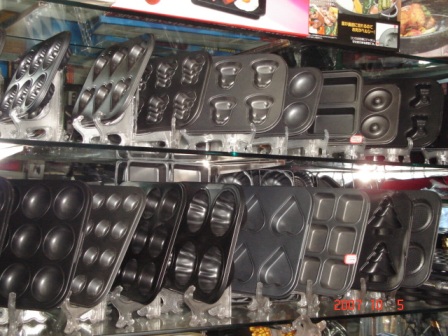This color photograph, taken inside a shop, features two glass shelves meticulously lined with baking trays and cake pans. The pans are all made of aluminum, exhibiting a uniform silvery charcoal gray hue. Each shelf holds eight molds: the top shelf showcases a variety of shapes including round pans, donut or mini bundt cake pans, and unique designs like one resembling a light bulb. The bottom shelf also presents an assortment of shapes—there are larger and smaller round tins, heart-shaped pans, square pans capable of housing six muffins each, and even molds shaped like Christmas trees. The detailed arrangement and diverse shapes of the baking trays give the display an organized yet dynamic appearance. Additionally, the upper part of the photograph hints at colorful appliance packaging, with a pink box that intriguingly features an appliance image with a fried egg.